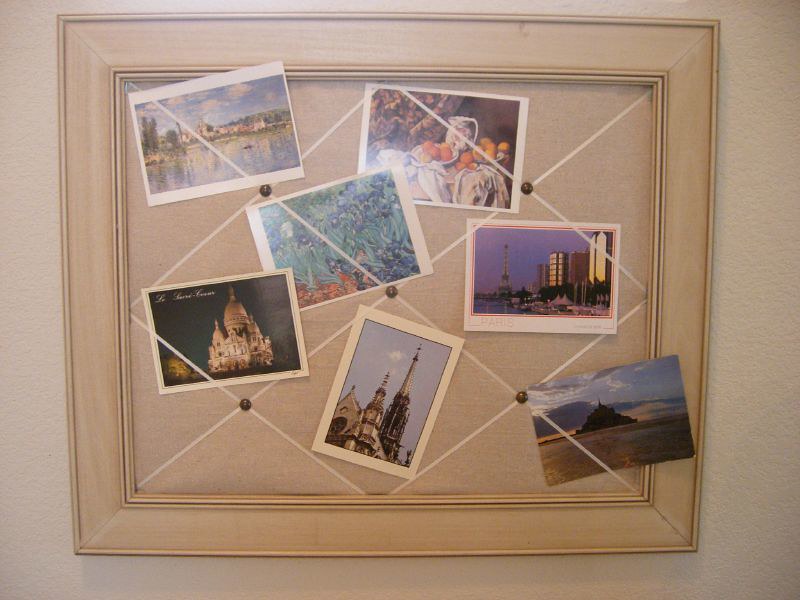The image showcases an ivory-finished wood organizing board, prominently displayed on a light cream-colored wall. The board features a thick, elegant frame that encloses a padded cloth background. This background is intricately adorned with a crisscross pattern of white ribbons, secured at intersections by brown upholstery tacks, forming a series of diamond shapes.

The ribbons function as holders for various postcards and photos, allowing them to be easily slid in and out. There are seven postcards visible, each capturing a different subject. Among them is a reproduction of Van Gogh's "Irises" painting with its vibrant purple flowers. Another painting depicted features oranges, potentially a still life. Additionally, there is a Monet landscape in the upper left corner, known for its serene and impressionistic style. Other postcards showcase landmarks such as the Eiffel Tower, various cathedrals, a beachside town, and possibly a mossy landscape. The colors in the postcards predominantly feature greens, blues, and earth tones, adding to the eclectic and visually rich display of this organizing board.